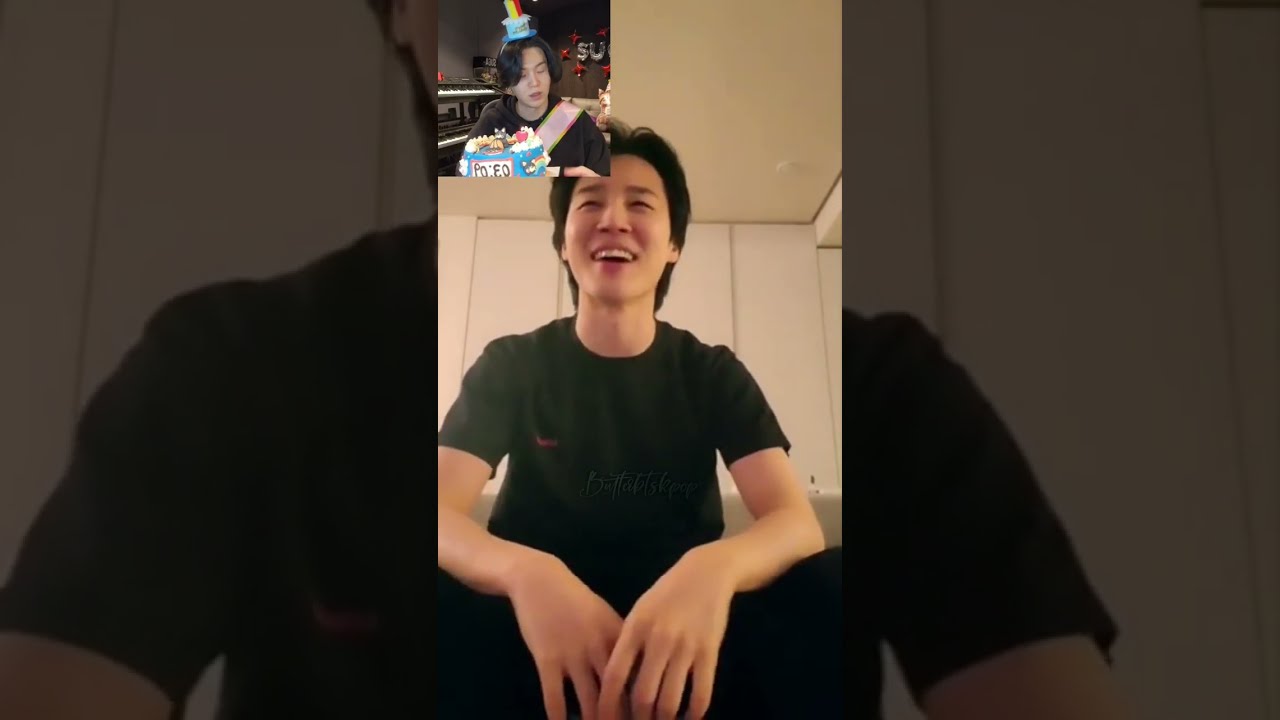The image depicts a young Asian man sitting down, dressed in a black t-shirt and black pants, smiling as he seemingly reacts to a video. Behind him is a neutral, cream-colored wall with a white ceiling that contains a smoke detector. In the top left corner of the image, there's a smaller inset showing another young Asian man wearing a whimsical blue cake hat with a rainbow on it. This man is seated in a decorated setting featuring star balloons and balloons that spell "SU," with several keyboards in the background. He is in front of a blue-frosted cake that has a gray cat figurine with a rainbow on it, and text that appears to read "P-O;E-O." The overall scene suggests the main subject is enjoying a video call or reacting to the content involving a light-hearted celebration.